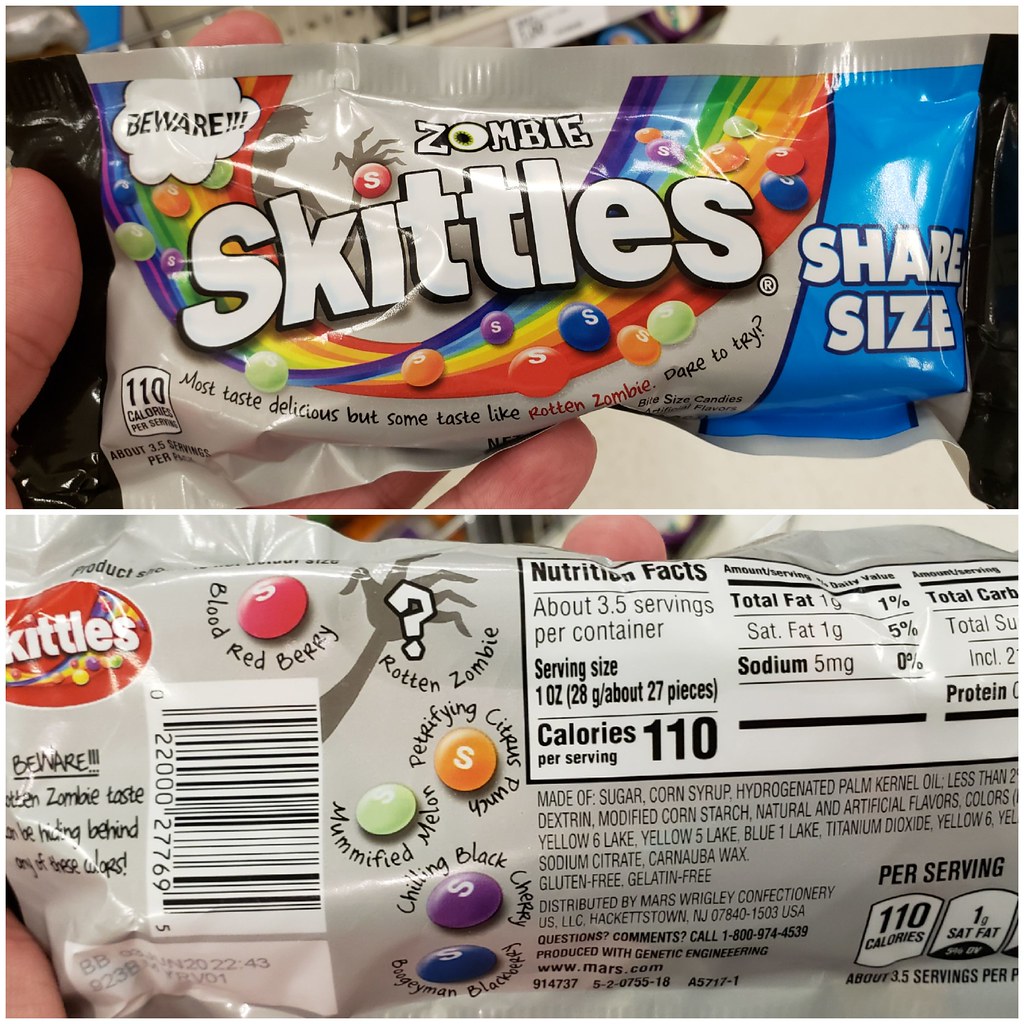The image comprises two rectangular, landscape-oriented photographs stacked vertically. The top photograph is a close-up of a "Zombie Skittles" share-size bag, prominently displayed in someone's hand. The packaging features the word "BEWARE" on the left-hand side, accompanied by an illustration of a zombie, creating an eerie Halloween-themed vibe.

The bottom photograph captures the back side of the same Skittles bag, also held by the same hand. The text on the left side reads, "BEWARE, ZOMBIE TASTE can be hiding behind any of these wraps," hinting at the surprise element in the flavors. The back of the bag also lists the different Skittles flavors associated with specific colors and includes nutritional facts and an ingredient list neatly printed underneath. The photos together provide a comprehensive view of the product's front and back packaging details, highlighting its playful and spooky theme.